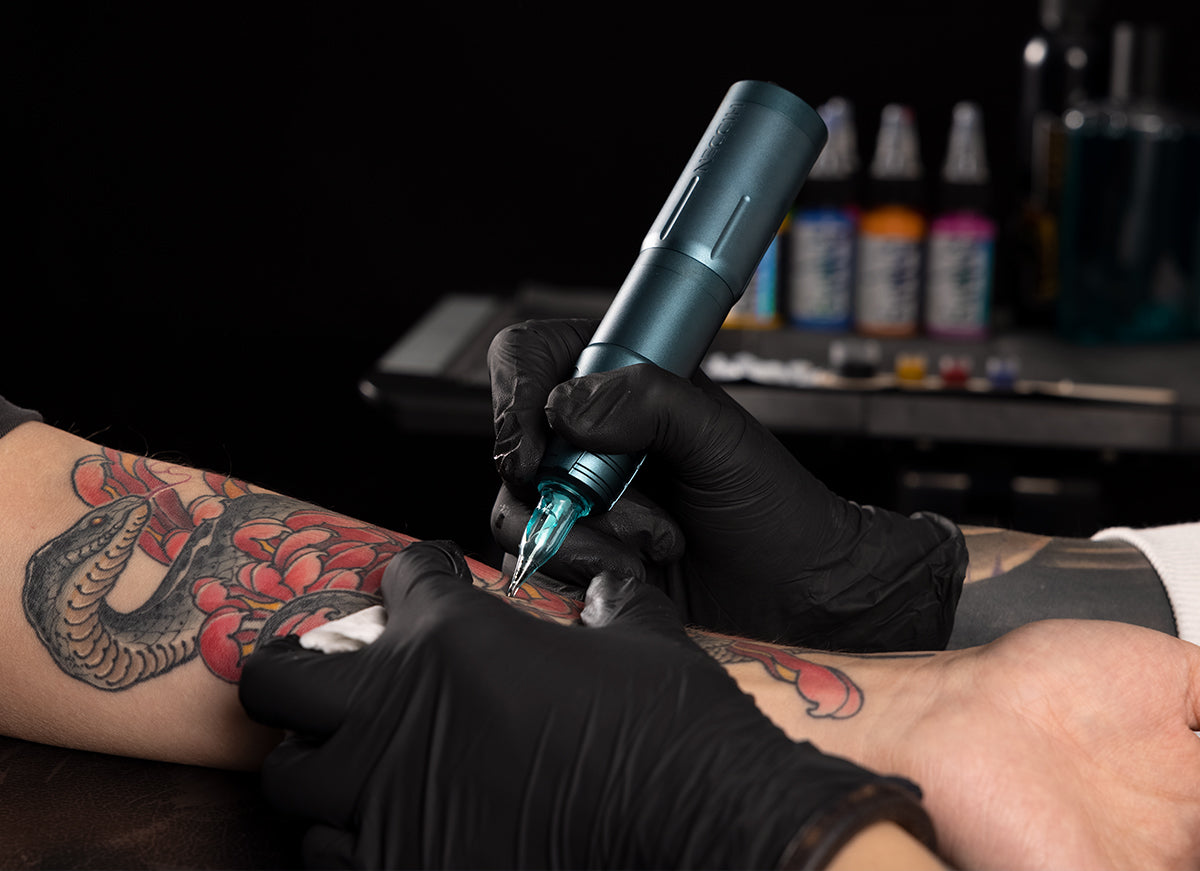The close-up photograph captures the process of a tattoo being applied to the inner forearm of a person with light-colored skin, whose arm is positioned palm up and extends from the left side of the image across the middle to the lower right corner. The artwork being etched is an intricate design featuring a black snake emerging from vibrant red-petaled flowers. The tattoo artist, whose presence is indicated only by their black latex-gloved hands, is diligently working on the forearm. One gloved hand is stretching the skin taut to ensure precision, while the other operates a large metallic blue and silver tattoo needle gun. The artist's left hand grips a paper towel, likely to clean excess ink or blood. In the dim background, a black cart stacked with an array of colorful ink bottles and various tattooing tools can be spotted, emphasizing the professional setting.